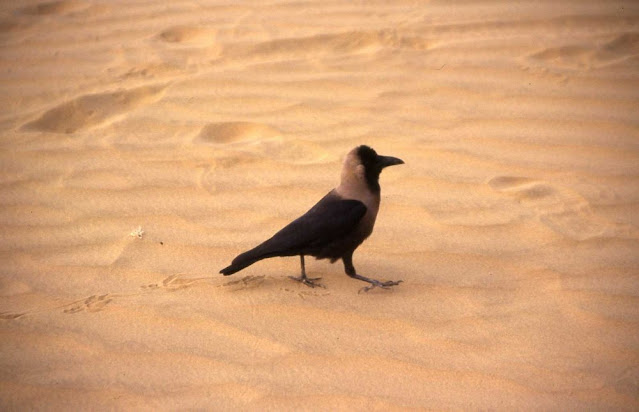The image features a bird prominently centered, walking across a vast expanse of sand. The sand in the background is mostly undisturbed, save for a few human and bird footprints scattered throughout. The bird itself has a predominantly black body, with its feathers darkening to black around the neck and face, and transitioning to lighter gray or brown near the back of its head. Its beak and face are also black. The bird is posed as if mid-step, with its right leg extended forward and its left leg planted in the sand. The bird’s tail feathers, also black, point straight back. The sand around the bird shows slight pitting and indentations, including slash marks and circular impressions.